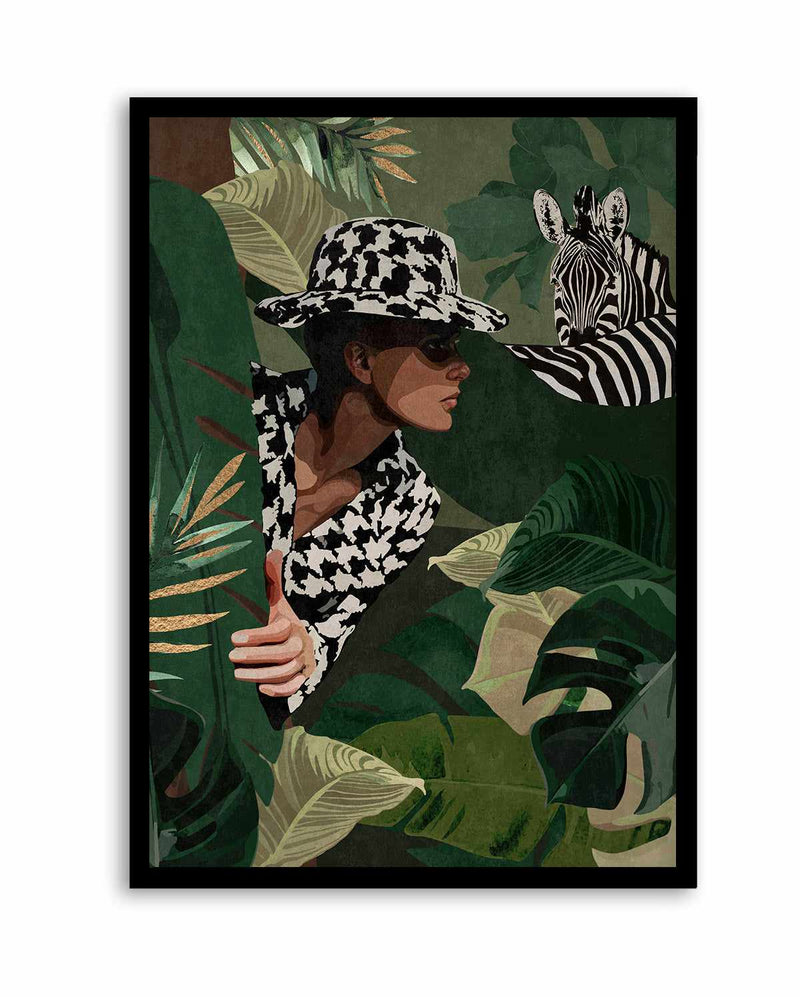This painting is a vertically framed, digital artwork that captures an enigmatic scene deep within a lush jungle. Dominated by vibrant greens and diverse foliage, the setting is replete with palm trees and the distinct presence of a zebra situated in the background. The zebra, displaying its iconic black and white stripes, is turned to face a solitary figure positioned towards the right of the frame.

The central figure, a woman of white complexion—or possibly a femininely built man—exudes a blend of mystery and elegance. She showcases a striking profile with a well-built, graceful neck, adorned in a black and white camouflage print ensemble. Matching both her button-down shirt with a V-neck and a hat reminiscent of either a bucket or safari style, her attire blends seamlessly with the jungle’s wild aesthetic. The shirt's top buttons are casually undone, adding to her intriguing appearance.

She dons dark sunglasses, further enhancing her air of mystique, and is seen leaning out from behind a brown tree trunk, hand resting on either a tree or a leaf. The artist has masterfully painted her looking towards the right, almost in a tranquil contemplation, amidst the dense foliage. This image, combining elements of both natural beauty and human intrigue, creates a captivating jungle tableau.